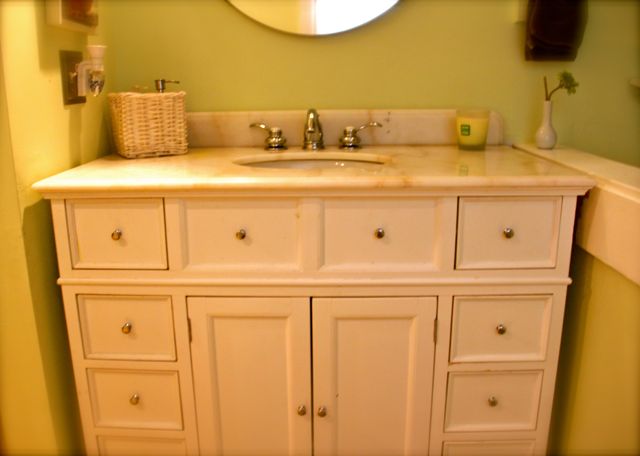A detailed image of a bathroom vanity set in a lime green room. The lime green walls have an unpleasant, somewhat "pukey" hue. The bathroom vanity is white, featuring a creamy countertop with black and brown marbled accents. The vanity is equipped with two center doors leading to the under-sink area, framed by a false drawer above and two sets of four drawers, each adorned with small metal knobs. The white paint on the vanity appears to be applied thickly, suggesting multiple layers.

On the right side of the vanity, there's a half-wall with a light tan Formica cap forming a rectangular frame. Atop this half-wall rests a vase containing a blue chrysanthemum. Above the half-wall, there's a blurry towel rack with two towels hanging from it. The round mirror hanging above the vanity reflects the room's somewhat somber ambiance.

To the right side of the sink sits a yellow candle in a clear glass container, featuring a green label. On the left side, there is a light-colored wicker basket, approximately six inches by six inches, containing a hand soap pump dispenser and another clear bottle behind it.

A cream and clear fragrance diffuser is plugged into the wall, contributing to the decor and atmosphere. The sink is equipped with chrome hardware, completing the bathroom's eclectic, albeit unsettling, design.